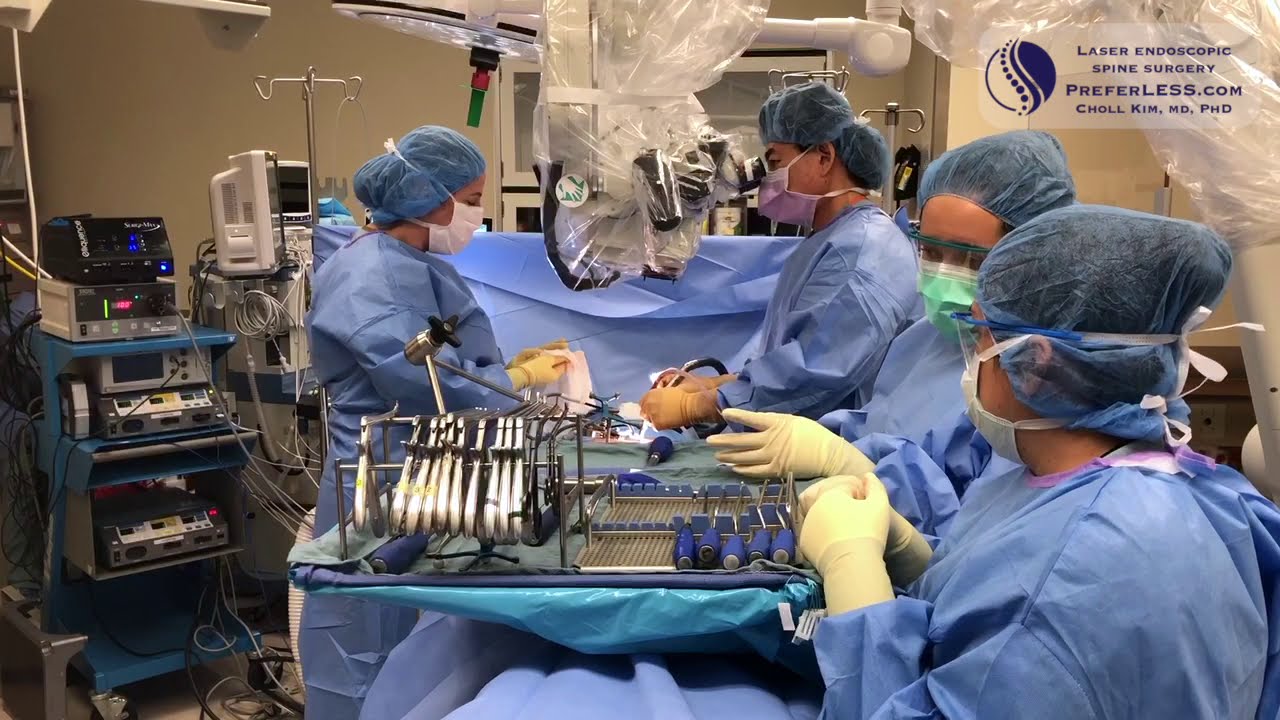This promotional color photograph showcases a laser and endoscopic spine surgery in progress, led by Chol Kim, MD, PhD, from Referralist.com. The image captures a well-equipped surgical room with four medical professionals—dressed in blue surgical scrubs, blue hairnets, white surgical masks, and yellow gloves—engrossed in their tasks. They are gathered around a central surgical table draped with blue sheeting. 

In the foreground, a tray crowded with various surgical instruments is visible, indicating preparation for a complex procedure. To the left, several pieces of medical equipment, including an IV pole with no attached bags and an electrical monitoring system, stand ready to assist in the operation. Although the patient remains out of view, the meticulous setup and focused activity suggest a spine surgery is underway. Above the scene, a piece of equipment hangs from the ceiling, encased in protective plastic, while a circular logo on the top left corner of the image reads "Laser Endoscopic Spine Surgery Referralist.com Chol Kim, MD, PhD," underlining the promotional nature of the photograph.